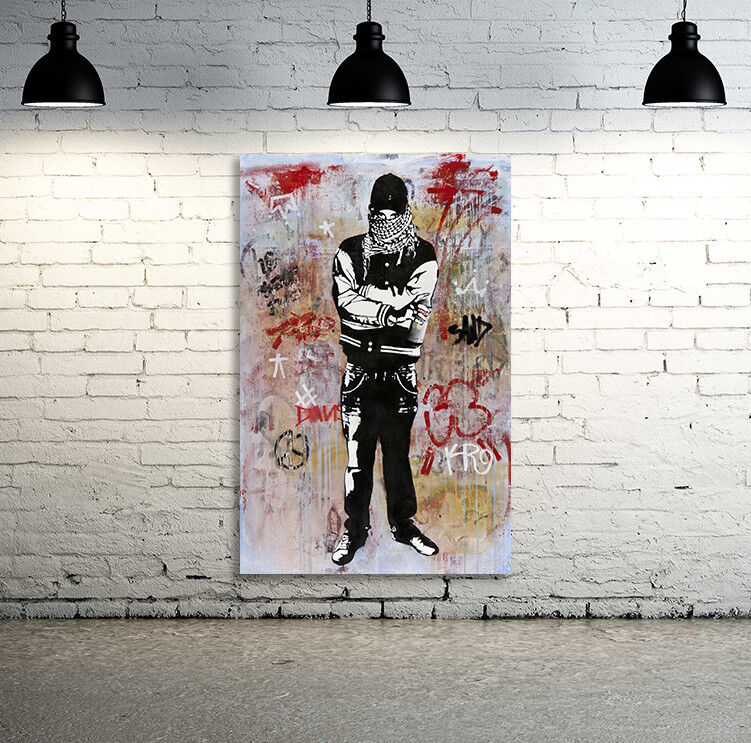The image showcases a Banksy-style piece of artwork mounted on a white brick wall under three black ceiling lamps, evenly spaced. Central to the artwork is a painting of a young man rendered in black and white. He is depicted in a defensive stance with arms folded. He's dressed in a baseball-style jacket with white sleeves and a black body, dark jeans, a belt, and white sneakers. A black beanie and a white scarf conceal his mouth and nose, revealing only his eyes, which convey a sense of hostility. The background of the canvas is a chaotic mix of graffiti symbols and tags in red, black, and tan shades. Notable elements include a black peace sign, an upside-down white crown, and the name "Dave" along with the initials "KR." The setting appears modern, with a rough gray floor visible beneath the canvas.